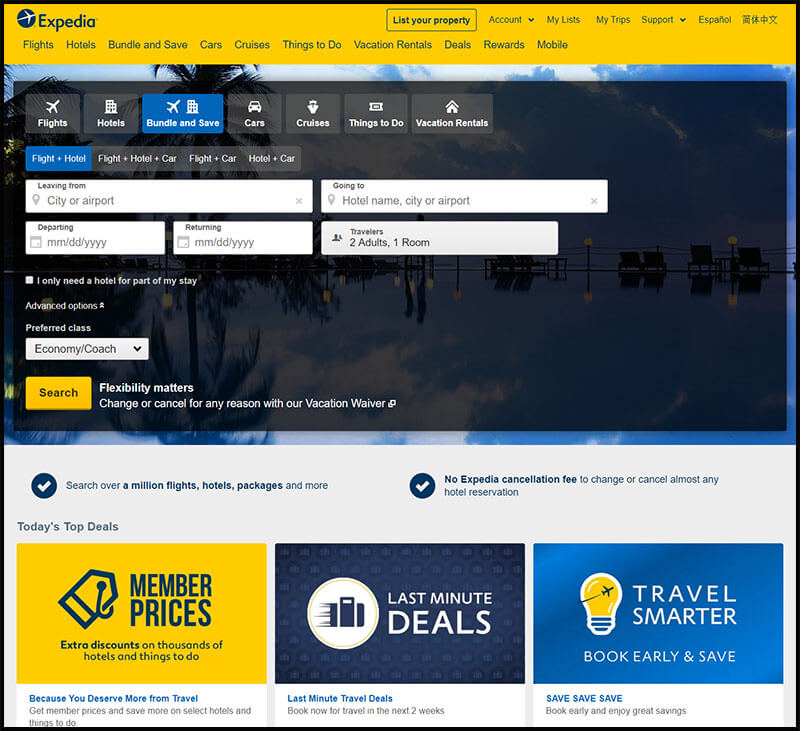This screenshot from Expedia's website showcases the 'List Your Property' option at the top of the page, inviting property owners to register their listings. The interface displays various navigational tabs including 'Accounts', 'My List', 'My Trip', 'Support', and language options ('Español', and 'Chinese'). The main section features Expedia's core services such as 'Flights', 'Hotels', 'Bundle and Save', 'Cars', 'Cruises', 'Things to Do', 'Vacation Rentals', 'Deals', 'Rewards', and 'Mobile'.

Central to the screenshot is a grayed-out background image partially obscured by an active pop-up window. This pop-up highlights the 'Bundle and Save' option, aimed at users looking to book both flights and hotels together. The booking form includes fields for departure and destination locations and points of travel, along with departure and return dates. Users can also specify if they need a hotel for part of their stay. Advanced options let users choose their preferred flight class (e.g., Economy/Coach).

Additional features include the flexibility to change or cancel bookings at any time through the vacation waiver program. Below the booking form, three highlighted blocks are visible: a gold block promoting 'Member Prices', a navy block for 'Last Minute Deals', and a blue block with a yellow bulb icon encouraging users to 'Travel Smarter'. There's an assurance of no Expedia cancellation fees, though the process may require searching through numerous flight and hotel options to find the best deals.